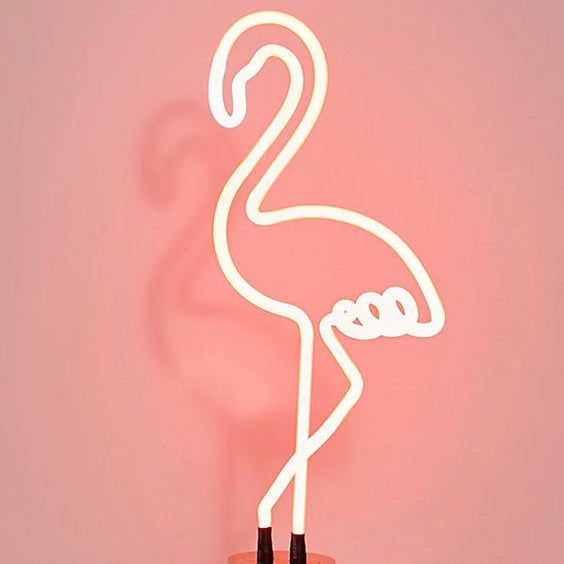The image features a striking neon LED sign of a pink flamingo at the center, its vibrant shape created by bright, fluorescent pink light. The flamingo is depicted with a long, curved neck and one leg crossed, standing as if on sockets that power the sign. The background is a solid, darker pink, providing a stark contrast to the illuminated bird. Shadows cast by the neon flamingo fall to its left and behind it, adding depth to the picture. This stylish and eye-catching piece could easily be found in a high-end boutique, a chic shopping store, or as a decorative feature in the home of a teenage girl or someone with a keen interest in pink flamingos.